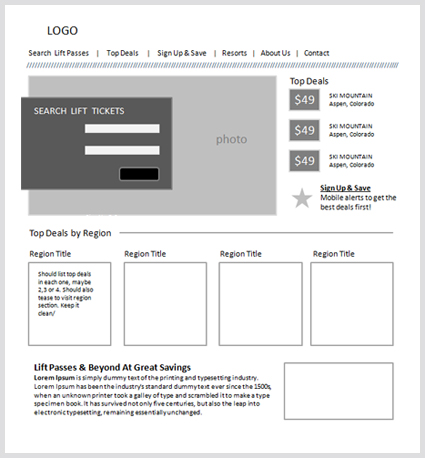The image is a screenshot of an advertisement, featuring a white background with a gray border along all four edges. In the top left corner, a logo is prominently displayed in large black font. Below the logo, a horizontal navigation menu appears in black text, listing the following options: "Search," "Lift Passes," "Top Deals," "Sign Up and Save," "Resorts," "About Us," and "Contact."

Under the menu, a row of tiny black dashes separates it from the content below. A gray rectangle follows with the word "Photo" in a slightly darker gray font positioned inside. Overlaying this gray rectangle is a darker gray box, within which "Search Lift Tickets" is written in white font. Below this, two white rectangular buttons and a black button are arranged vertically.

On the right side of the image, the text "Top Deals" is written in black font, with the following deal listed multiple times: "$49, 5k Mountain, Aspen, Colorado." The same deal description repeats twice more in identical presentation.

Toward the bottom, a prompt to "Sign up and save mobile alerts to get the best deals first" is shown. To the left of this text sits a gray five-pointed star, completing the visual layout.